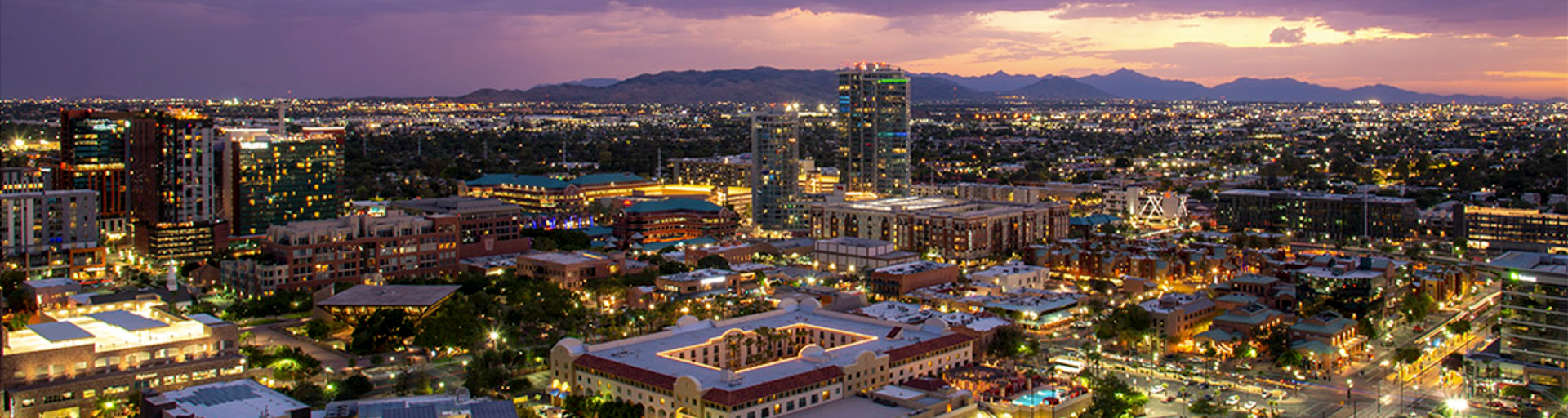This photograph captures an aerial view of a sprawling cityscape at dusk, beautifully illuminated by countless lights. The city is densely packed with buildings of various sizes and shapes, filling nearly three-fourths of the image. Scattered trees add a touch of greenery, while a prominent road can be observed on the right side. The sky above is a mesmerizing palette, transitioning from rich purples and pinks on the left to golden and red hues on the right, indicative of the setting sun. A break in the clouds allows streams of yellow sunlight to cascade through, casting a peaceful and heavenly glow over the scene. The backdrop of mountains beneath the vibrant sky further enhances the serene beauty of this evening cityscape.